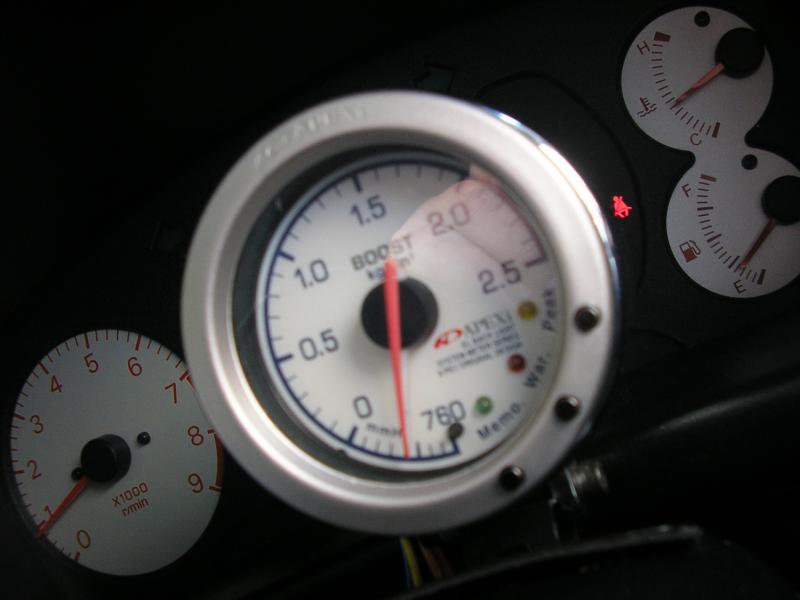A detailed and focused image showcases the control panel of a vehicle, prominently featuring several gauges. The central gauge, larger than the others, is labeled "Boost." Below this label is a red dial with a scale extending around 270 degrees from the bottom. The scale starts at 760 and progresses through 0.5, 1, 1.5, 2, and 2.5. Around the rim of this gauge, there are LEDs labeled with text: a green LED marked "Minimal," a red LED labeled "WAT" (though the text is somewhat unclear), and a yellow LED labeled "Peak." There is also a red logo accompanied by indecipherable text next to this gauge.

To the left of the central gauge is a smaller gauge featuring a red hand, a white face, and red numerals. This appears to be a tachometer, with markings in intervals of 1,000 revolutions per minute (indicated as "by 1,000 R/min"), where a reading of 1 equates to 1,000 RPM.

To the right of the central gauge, there is a double gauge. The upper section of this gauge has an icon indicating temperature, with readings ranging from 'C' (cold) to 'H' (hot). Below it, the lower section features an icon of a gas pump and displays fuel levels from 'E' (empty) to 'F' (full). Positioned between the temperature and fuel gauge and the central boost gauge is a red seatbelt icon, which is illuminated.